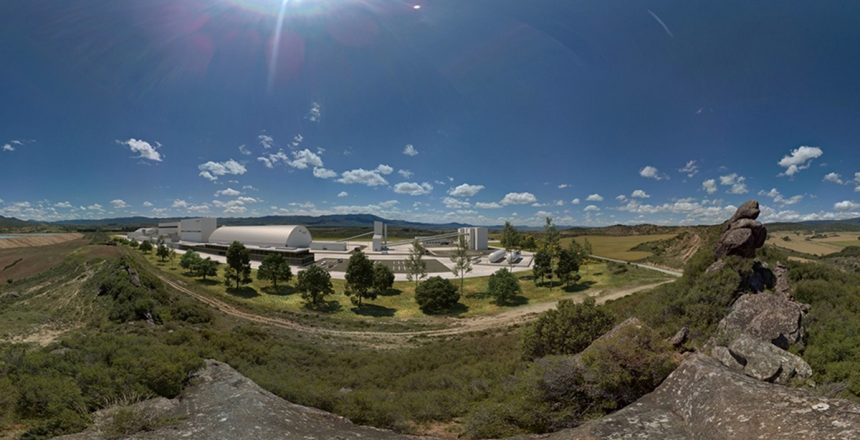The image is a wide-angle shot of a rural landscape, taken in daytime with the sun shining bright in a clear, dark blue sky dotted with a few white clouds. The foreground features gray rock formations, which lead into a scene that appears slightly distorted, as if viewed through a curved lens. At the heart of this landscape is an industrial or manufacturing plant, situated on a large concrete area resembling a vast parking lot. The plant comprises various steel-colored structures, including cylindrical silos, square buildings, and white tankers, with some wires and utility activities evident. This industrial complex is encircled by a roadway forming a loop around it, beyond which lies a well-maintained garden with neatly spaced, lush green trees. Surrounding the entire scene are open fields and desert-like terrain that stretch out toward distant hills or mountains, enhancing the sense of isolation and rural charm in this picturesque setting.